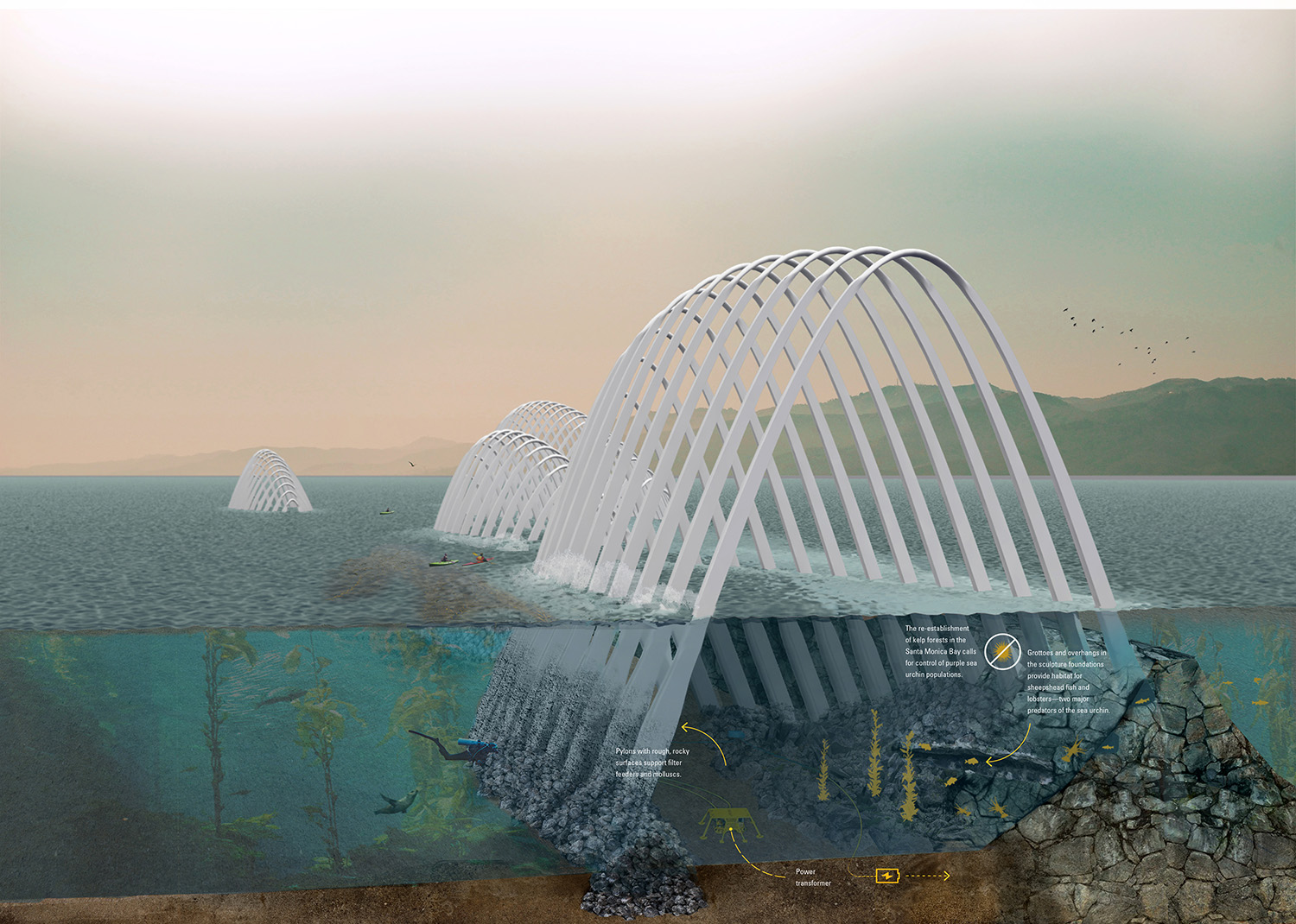The image is a detailed digital drawing in landscape mode, depicting a series of white arch-like structures submerged in the ocean. The forefront features the largest of these arches, standing approximately 50 feet above the water and extending another 30 feet into the ocean floor, secured by rocky, mortared bases. This large arch is followed by three smaller, similar structures in the background, all of which appear to be constructed from a metallic white material. The setting includes a scenic backdrop of mountains in various shades of green and yellow, under a sky tinged with hazel gray and light yellow-green hues. The ocean itself is depicted with blue and green waves, teeming with underwater life including divers, seals, and various fish. On the ocean's surface, three people are seen kayaking near the arches. Additionally, there are elements like a power stabilizer labeled in the image and other environmental interpretations, such as filter feeders and habitat formations for sheephead fish and lobsters, which help control the purple sea urchin populations. The background also shows a clear open sea view with a couple of boats and a patch of birds flying near the distant mountains. This intricate diagram suggests these arch structures function both as artistic installations and ecological habitats, contributing positively to the marine environment.